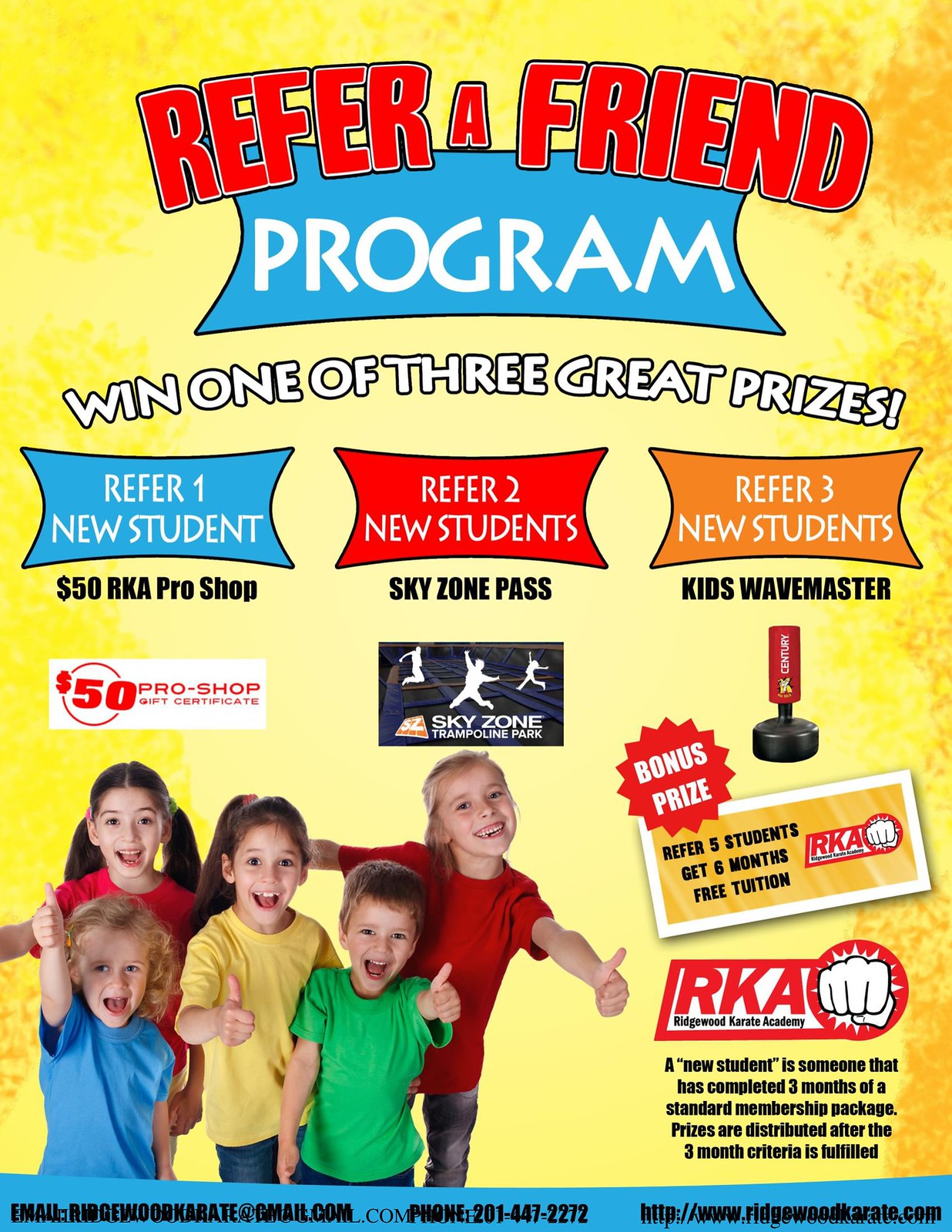The image is an advertisement with a vibrant yellow background and red lettering at the top that reads "REFER A FRIEND." Below this, within a blue curved rectangle with white font, it states "PROGRAM." Further down, it announces in white capital letters, "WIN ONE OF THREE GREAT PRIZES." The image also highlights various reward levels within differently colored rectangles: referring one new student earns a $50 RKA Pro Shop gift certificate; referring two new students yields a Sky Zone Trampoline Park pass; and referring three new students wins a Kids Wave Master. Additionally, there's a bonus prize mentioned on a red background, stating, "REFER FIVE STUDENTS, GET SIX MONTHS FREE TUITION," for the RKA Ridgewood Cotterotty Academy. At the bottom left corner of the ad, there’s a group of five cheerful children wearing brightly colored t-shirts, all smiling and giving a thumbs-up. An important note clarifies that a new student is defined as someone who completes three months of a standard membership package, with prizes distributed after this three-month criteria is fulfilled.